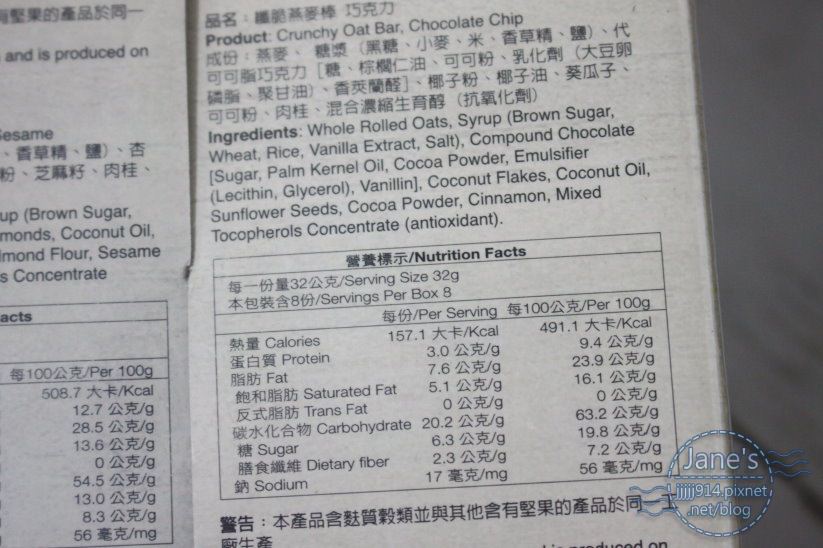The image features a detailed ingredient list printed in black text on a white cardboard background, showcasing both English and possibly Chinese or Japanese characters. The image shows two adjacent columns of information, with only the right column being fully visible. The left column is partially cut off and contains incomplete text. The central column lists ingredients for a "crunchy oat bar, chocolate chip," including whole rolled oats, syrup, brown sugar, wheat, rice, vanilla extract, salt, compound chocolate, coconut flakes, coconut oil, sunflower seeds, cocoa powder, cinnamon, and mixed concentrate. Below the ingredient list, a section titled "nutrition facts" provides details about calories, protein, saturated fat, trans fat, carbohydrates, sugar, dietary fiber, and sodium. At the bottom right, a circular logo reads "Jane's," with the website "jjjjj914.pixnet.net/blog" printed beneath it. The background beyond the ingredient list is indeterminate.